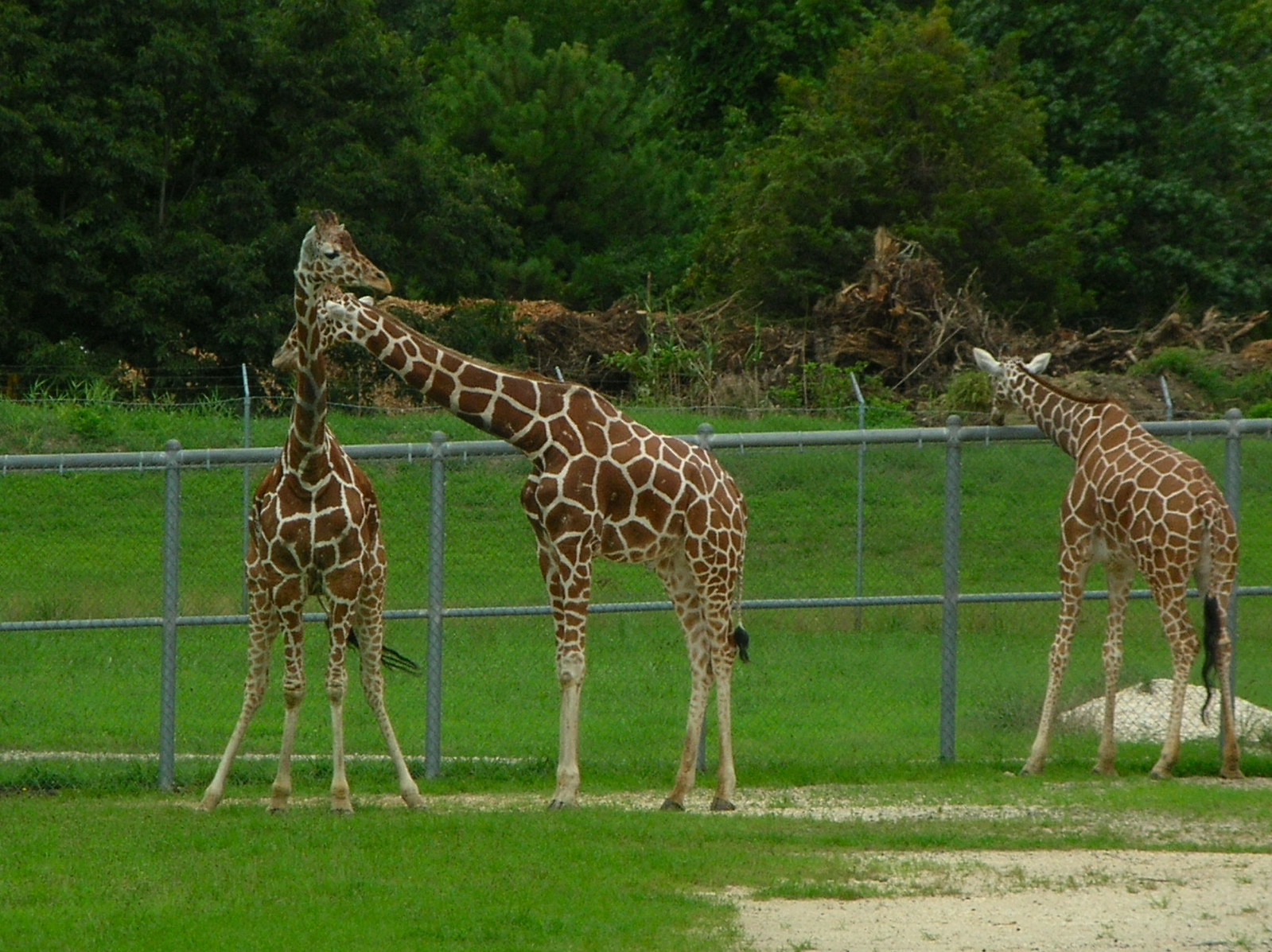In the image, three tall giraffes stand majestically within a fenced area, surrounded by lush green grass. The giraffes are predominantly yellow and orange with a striking pattern of white lines creating a mosaic of large orange tiles on their long necks and torsos. Their legs are white at the bottom, gradually transitioning into their patterned bodies. One of the giraffes, which seems younger and shorter than the others, leans its head over a gray chain-link fence, appearing to be interested in the grass beyond. The two taller giraffes are engaged in a playful interaction, with one gently touching the neck of the other. The background is a mix of verdant tall trees interspersed with areas of dead orange bushes, providing a vivid contrast. Beyond the immediate fence, a secondary fence runs parallel, reinforcing the secure area. Small details like the giraffes' black-tipped tails and the concrete patches on the ground contribute to the scene's intricate realism. This peaceful moment captures the essence of wildlife in a protected setting, with nature unfurling both behind and within the fenced enclosure.